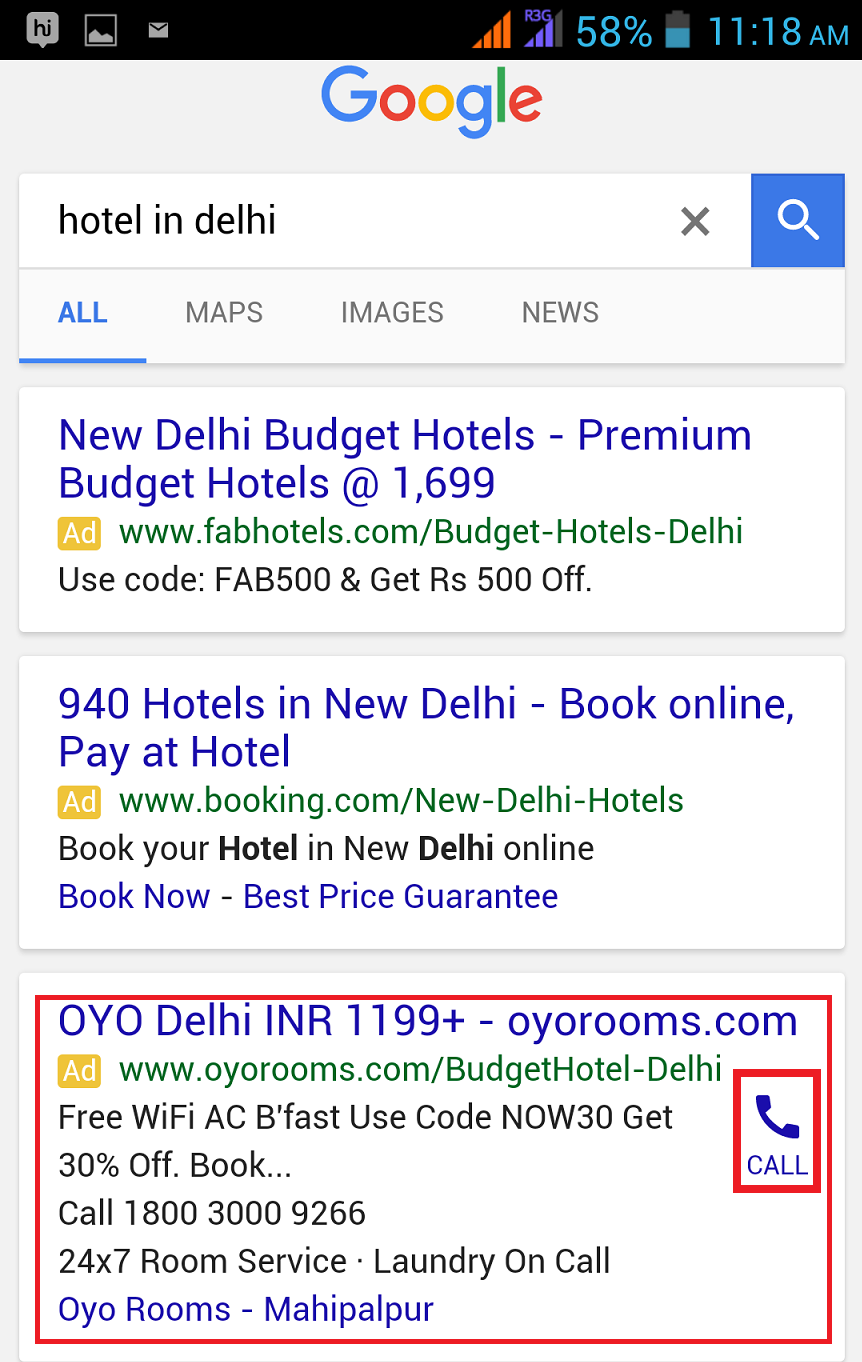Here is a detailed and cleaned-up caption for the image:

---

This image is a screenshot of a Google search on a cell phone. At the top of the screen, there is a black status bar displaying various icons and information. From left to right, the bar features a speech bubble icon with "HI" inside it, an image icon, a mail icon, and indicators for signal strength—one in red and another in a bluish-purple hue. The battery icon is teal and shows the level at 58%. The time is displayed as 11:18 AM.

Below the status bar, the Google logo is prominently displayed above the search box. The search query entered is "hotel in Delhi." To the right of the search box is a blue search icon. Beneath the search box, there are category tabs: "All" (highlighted in blue), followed by "Maps," "Images," and "News."

The search results are listed below these tabs. The first result is for "New Delhi budget hotels," with a premium budget hotel option priced at $1699. The link is displayed in green, and there is a mention of using the code "FAB500" to get ₹500 off.

The second search result shows "940 hotels in New Delhi," with the option to book online and pay at the hotel. This result includes an ad symbol, a green link, and a description in black text, "Book your hotel in New Delhi online," along with a "Book now, best price guaranteed" message in blue.

The third and highlighted result has a red border and is for "OYO Delhi" with prices starting at INR 1199. The link provided is to oyorooms.com and features another ad symbol. Additionally, it advertises free WiFi, AC, and fast service. There is a promotion to use code "NOW30" for 30% off. The contact number, 1-800-3000-9266, is provided for booking, along with an offer of 24-7 room service and on-call laundry. The result concludes with blue text indicating "OYOrooms-M-A-I-H-I-P-A-L-P-U-R."

---